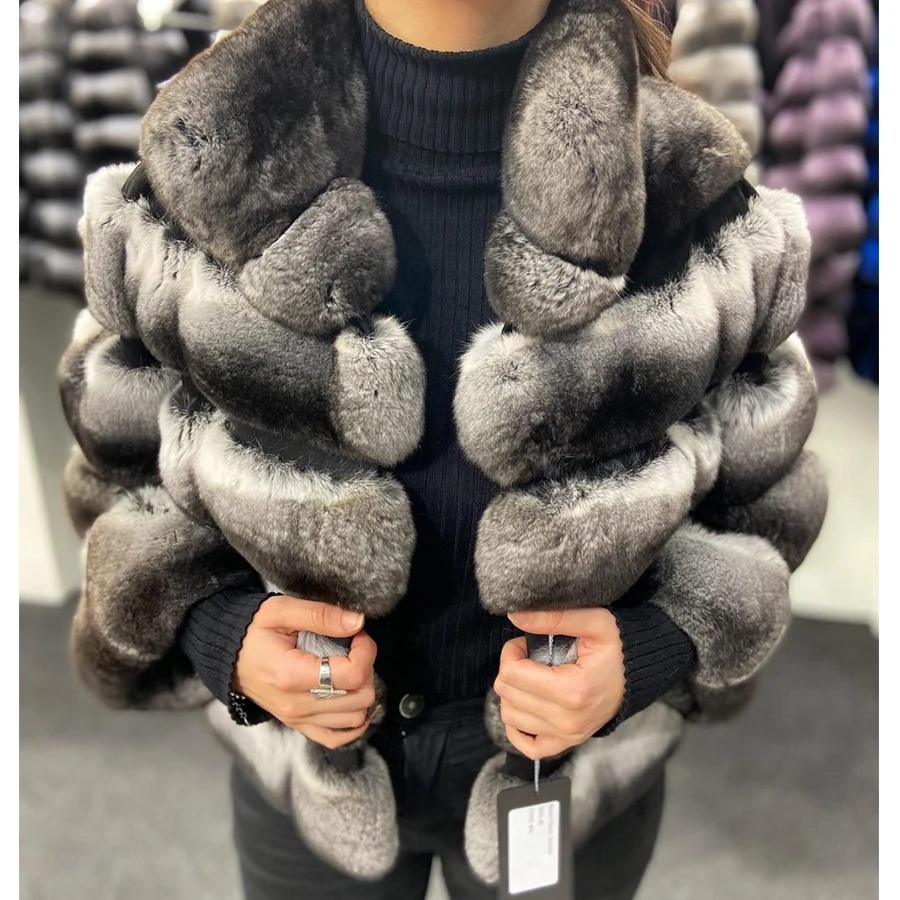In this square-cropped, indoor photograph, we see the torso of a woman from her neck to her upper thighs. She is dressed in a stylish winter ensemble, featuring a grey faux fur coat with a black tag that has a white label hanging from the lower left side near her left hand. The coat, which resembles a chinchilla or mink fur with a puffer jacket style, is layered over a black ribbed turtleneck sweater and paired with black jeans. The woman’s hands, adorned with manicured nails, are visible; she wears a silver ring on her left hand and another ring on her right index finger. The setting appears to be a fashion store, as evidenced by the similar fur coats hanging in the background. The floor is grey, further emphasizing the indoor environment. Only her neck and hands are visible; her face and feet are out of frame, but it's discernible that she is likely a white woman.